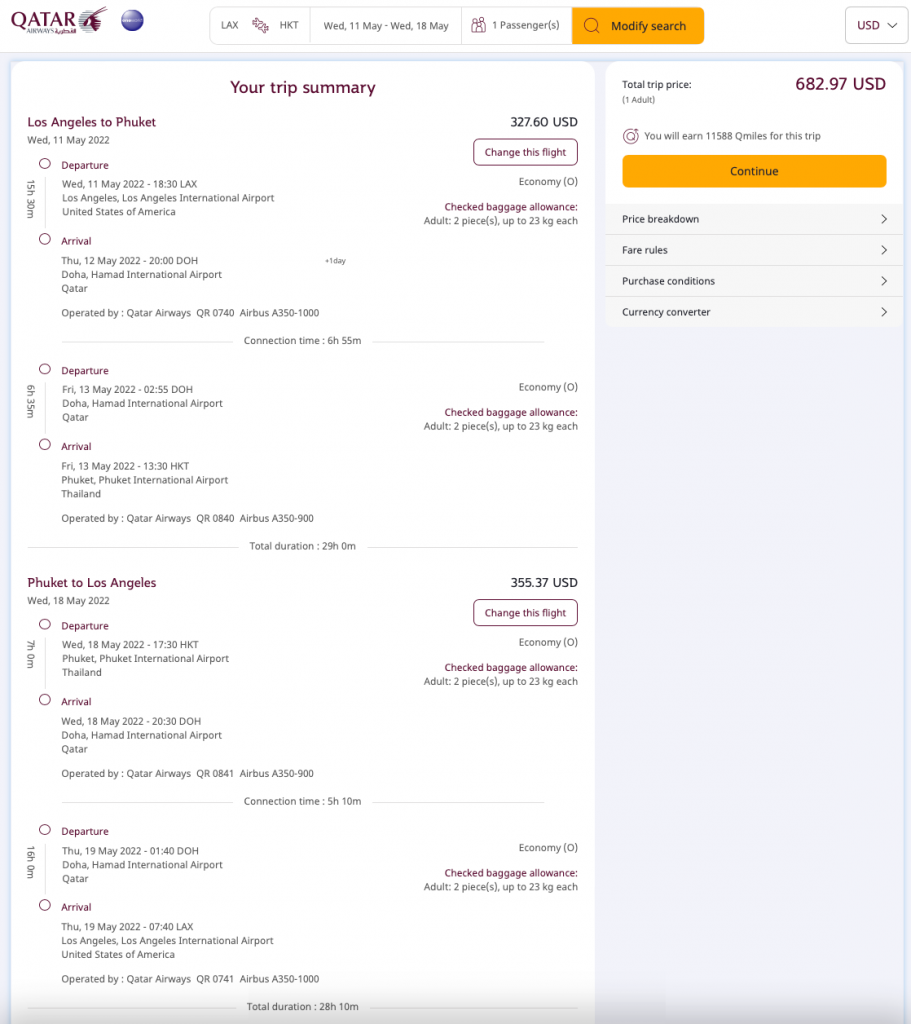The image depicts a webpage with tiny, difficult-to-read text, resembling a trip summary from Qatar Airways. The summary outlines a flight itinerary from Los Angeles to Phuket. Visible information includes the departure date from Los Angeles on May 11, 2022, and the return date from Phuket on May 18, 2022. The cost for the outbound trip is $327.60 USD, while the return trip is priced at $355.37 USD. The total cost for the round trip amounts to $682.97 USD.